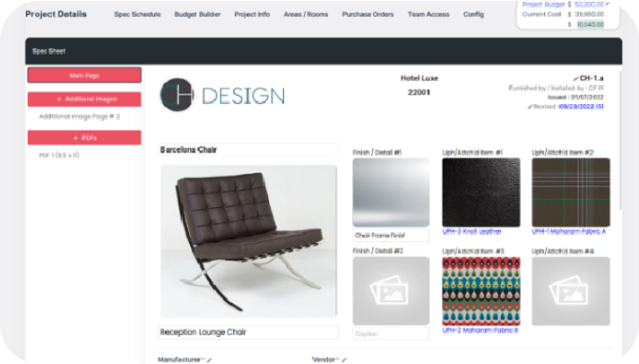**Title: Web Interface Overview for Project Management Platform**

**Description:**
This is a long panoramic screenshot showcasing a somewhat blurry web interface of a project management platform, making detailed text challenging to decipher. The interface is bordered on the left, right, and top by a gray border. At the top left, in black letters, the words "Project Details" are visible, suggesting a clickable menu. Despite the blurriness, the menu items appear to read, from left to right: "Spec Schedule," "Budget Builder," "Project Info," "Areas/Rooms," "Purchase Orders," "Name Access," "Config." On the far right within the gray border, there is a white box with blue text at the top that reads "Project Budget." Below it, a large dollar sign and a dollar amount are present but unreadable due to their small size. Beneath this, in black letters, it says "Current Cost," followed by another dollar sign and dollar amount, similarly unreadable, and a highlighted blue dollar tab beneath that.

The main content of the website features a long black bar at the top with some white text on the left that is too blurry to read. Below this bar are three red clickable boxes with white text. The top box on the far left reads "Main Page." Below it, another box with a plus sign seems to say "Additional Images," followed by "Additional Image Page 2." The final red box likely reads "Plus Pics," and below it is "Pics 1," followed by some numbers in parentheses that are unreadable.

Central to the image is a white background featuring a black circle with a blue "C" and a white "H" inside it, accompanied by blue capital letters spelling "DESIGN." To its right, black letters spell "Hotel Luxe 22," and below that, "22001." Further right is some text in black and blue, which is not legible.

Beneath the "HCH Design" section, the black text reads "Reception Lounge Chair." Below this description is a square image of a black leather chair on a white background, presumably the "Reception Lounge Chair." To the right of this image are two rows, each containing three potential design options for the chair. The top left design includes a gray and white pattern. The middle design in the upper row is predominantly black. The upper right option combines brown, white, and green plaid. In the lower left, there is a gray square with two scenery icons. The middle option in the lower row features a colorful pattern with white, blue, yellow, and green hues, though its exact design remains unclear. The lower right option is another gray square with a landscape icon.

At the bottom of the display, black text reads "Manufacturer and Vendor," but further details are cut off from view.